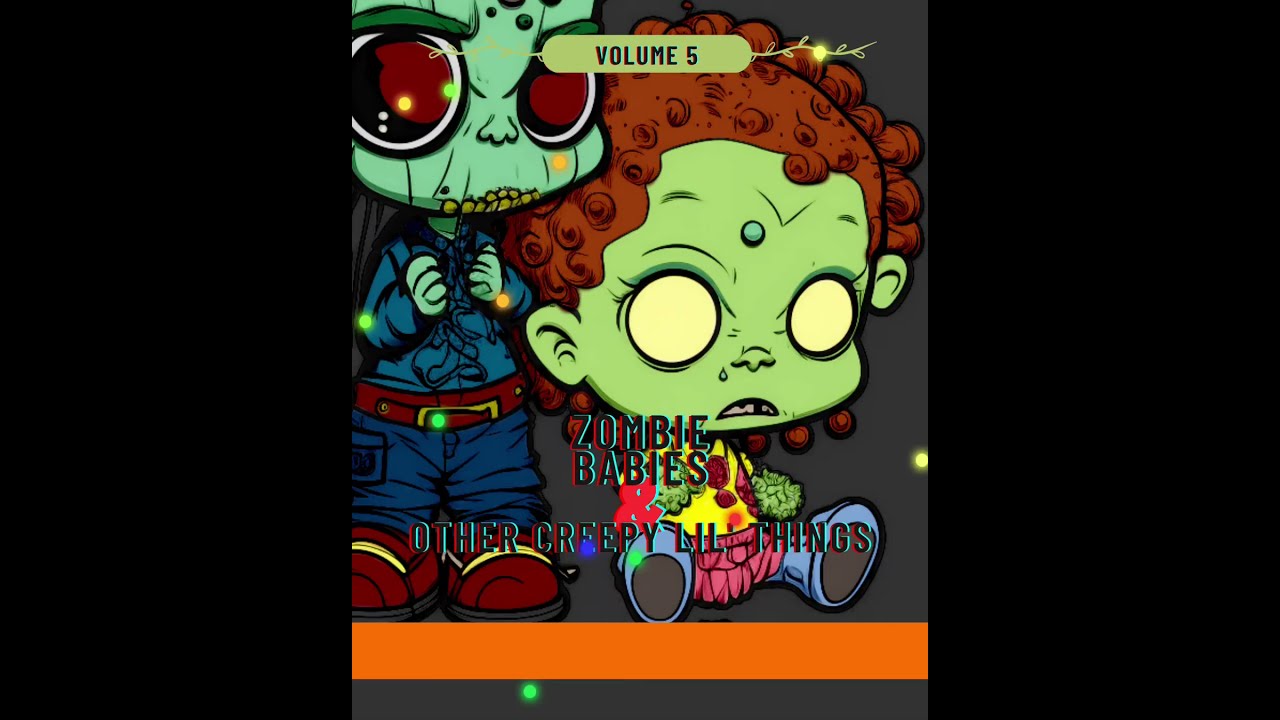The cover art, titled "Volume 5" in green lettering, prominently features two cartoonish zombie characters and the text, "Zombie Babies, Other Creepy Little Things," in multi-colored and black letters. The background is interspersed with sparkles and glowing lights in yellow and green hues, set against an orange band or stripe at the bottom of the image.

On the left stands a short, stubby zombie adorned in a blue shirt, little blue pants, and red shoes. This character has a green face with big red eyes, green fingers, and appears to be holding the collar of its jacket, giving off a slightly menacing or comical vibe with its rotten teeth and little nose.

To the right, a second zombie sits on the ground, characterized by a huge green head with big yellow eyes, a tear beneath one eye, and curly red-brown hair. This figure wears a yellow shirt, pink pants, and blue shoes, enhancing its baby-like, yet eerie appearance. Both characters exude a playful creepiness, perfectly fitting the "Zombie Babies" theme.